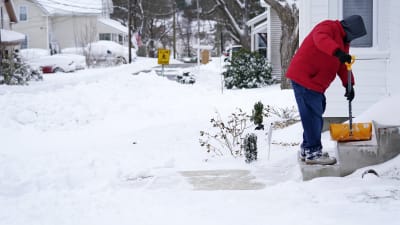The photograph captures a tranquil snowy scene in a neighborhood street blanketed entirely in white, with only a few hints of greenery poking through. On either side of the street, you see a couple of houses, some of which have cars in front, lightly dusted with snow. In the foreground on the right side, vividly standing out against the snowy backdrop, is a person dressed in a distinctive red coat with a black hood obscuring their face. They are shoveling their concrete front steps with an orange snow shovel. The person’s outfit also includes black gloves, blue jeans, and sneakers. The person is currently positioned on the first step of a three-step staircase, which is covered in snow except for the step they are standing on. The individual appears to be working on clearing the steps and has already made progress on part of the walkway leading up to the house. In the background, you can spot the side of a house with a window and more houses aligning the street, adding depth to this peaceful winter landscape.